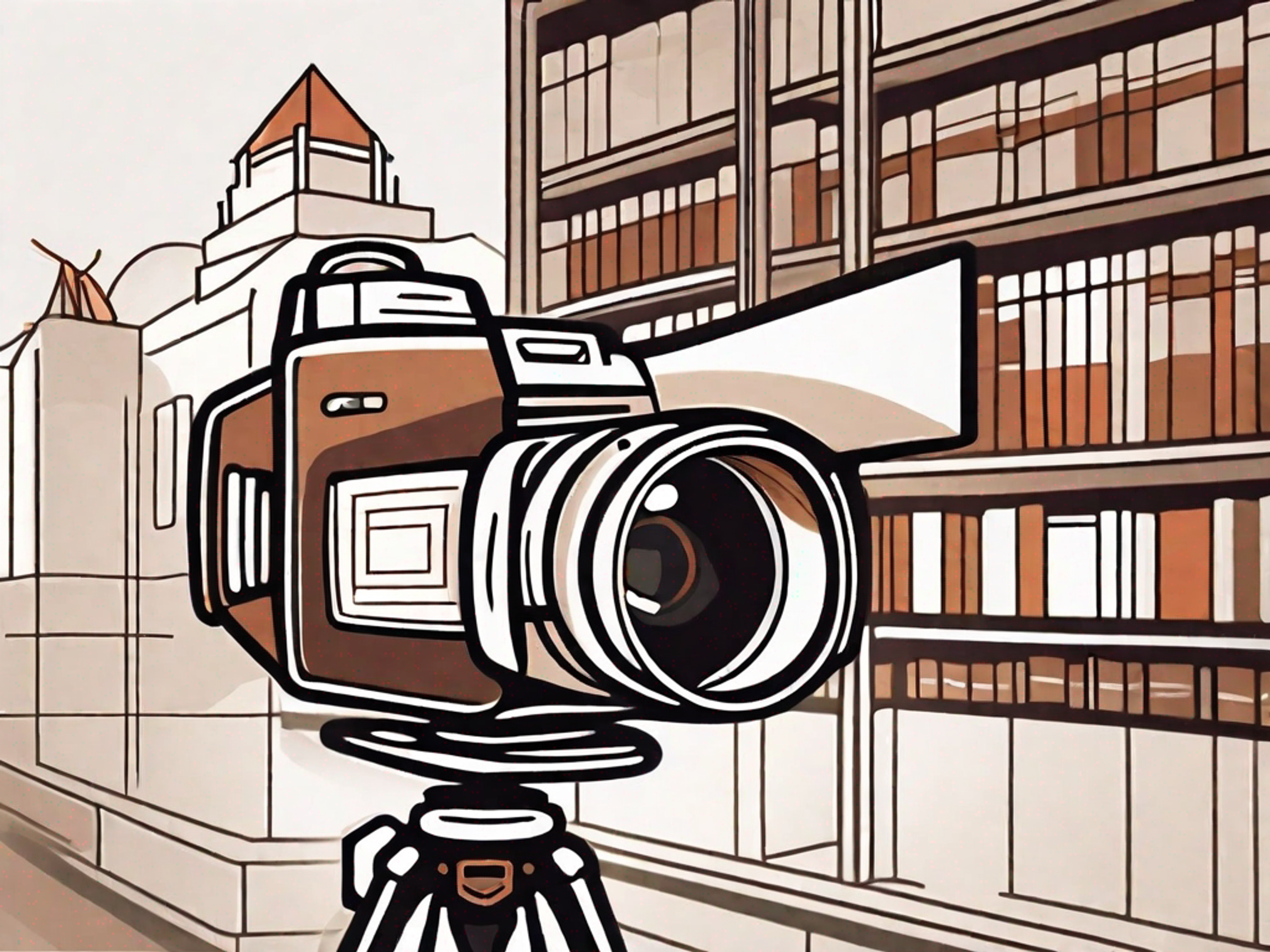The image is a stylized, minimalistic illustration depicting a scene set in a hybrid space that could be a library or a DVD storage facility. It primarily uses clean lines and a palette of brown, cream, and white to create a sense of structure and simplicity. At the center of the illustration is a large, professional medium format film camera, reminiscent of a Hasselblad, mounted on a sturdy tripod, exuding a cubic and hefty appearance. Surrounding the camera is an organized array of bookshelves laden with books or perhaps DVDs, characterized by various rectangular shapes. In the background, there's an architectural element with a distinctive triangular top, similar to the LA City Hall, adding a hint of grandeur and scale. The entire composition merges geometric shapes and minimalistic design, emphasizing a sense of organized chaos with its mix of visual elements.